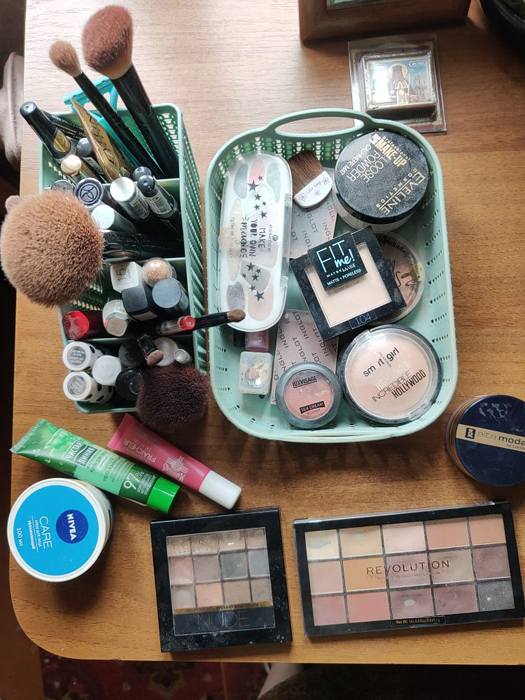An organized and detailed overhead view of a makeup collection displayed on a brown tabletop. The composition is a visual treat showcasing a vast assortment of makeup products. In the lower section of the image, two clamshell makeup palettes with clear lids stand out, readily awaiting a makeup brush for application. Positioned directly above these palettes is a green basket brimming with various beauty products, likely including foundations and other essential makeup items. Adjacent to this on the left, another green basket is neatly filled with application tools such as brushes, eyeliners, and potentially lip gloss applicators, hinting at a well-organized routine. Toward the lower-left corner, three distinct products catch the eye. One is a container with a blue lid, labeled 'Nivea,' and it sits beside a green tube and a pink tube with a white lid, each presumably filled with different beauty substances. This meticulous setup clearly represents the collection someone relies on regularly for their makeup needs.